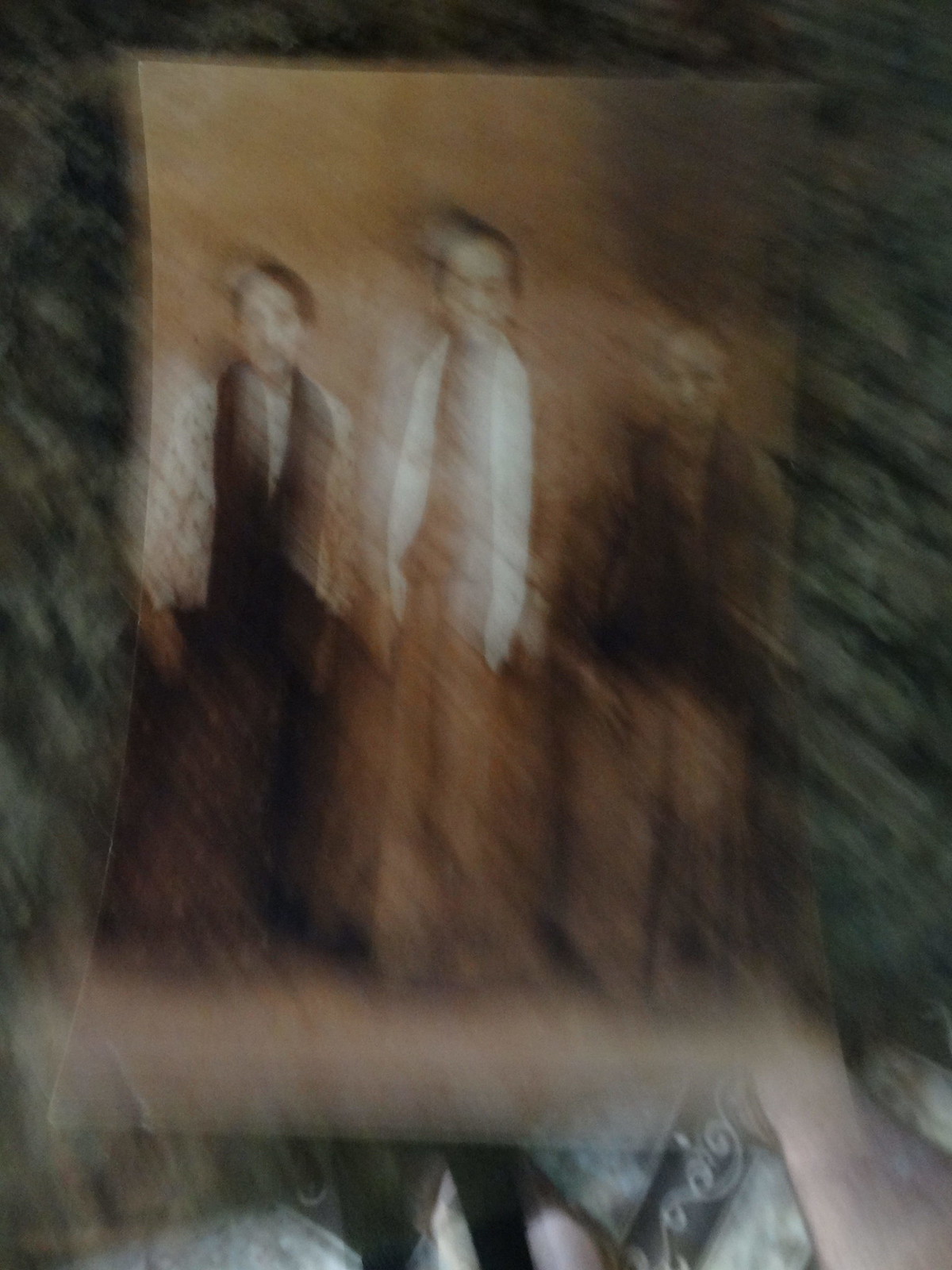A blurry, low-quality image shows three individuals in the center, with the tallest in the middle and the shortest on the right. Despite the fuzziness, the person on the left can be seen wearing a white top and a black scarf around their neck. The overall lack of clarity makes it difficult to discern facial features.